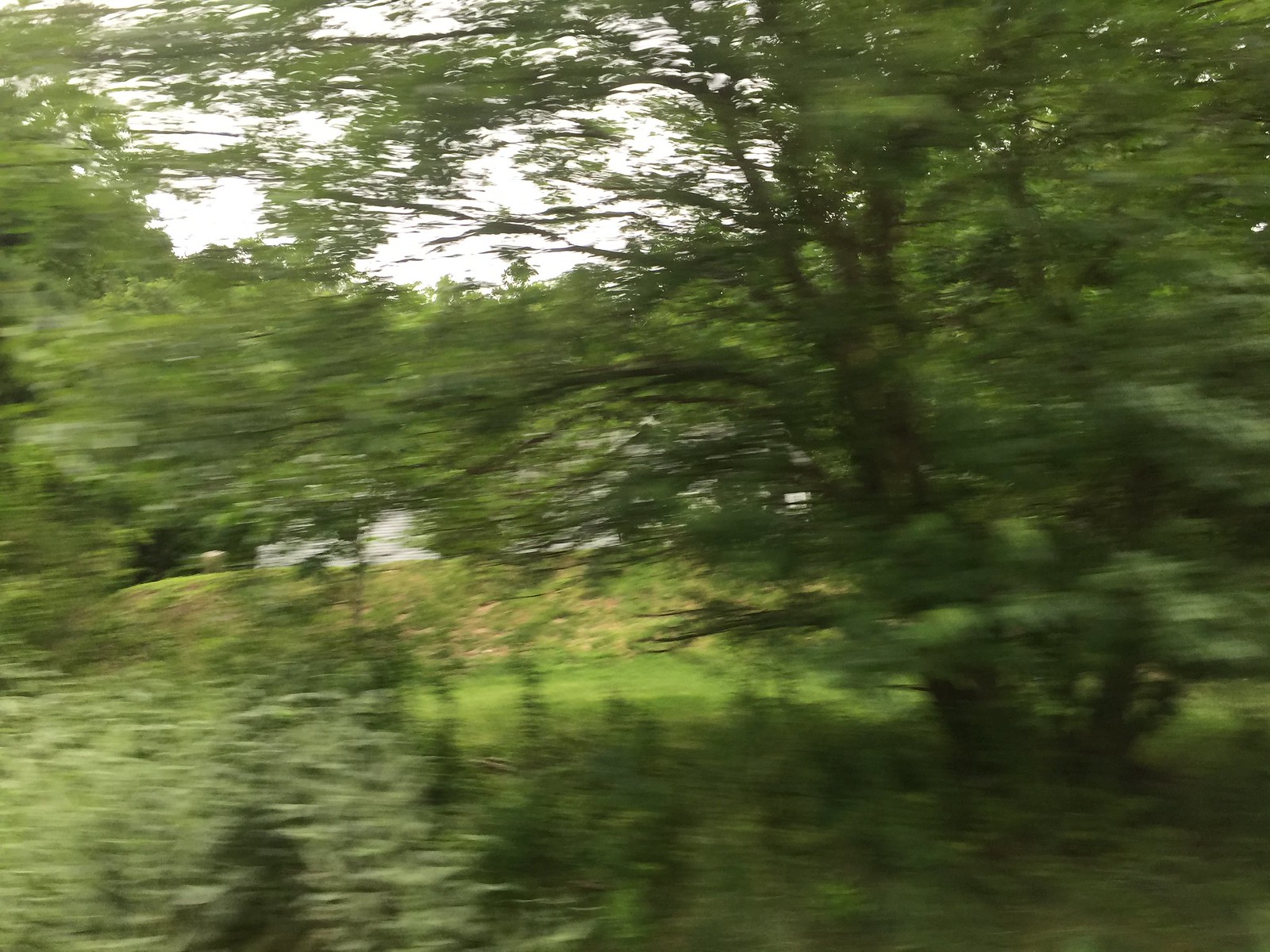This is a photograph taken during the daytime featuring a landscape of trees and lush green foliage. The image is notably blurry, with a shaken effect, as if the camera was moved while the picture was taken, contributing to a very skewed, indistinct appearance. The sky is partially cloudy with a grayish tone, and subtle lens flares indicate it was captured under sunlight. You can observe brown tree branches amidst the dense green leaves, as well as shadows cast by the trees on the ground. The ground itself is a mix of overgrown green and patches of dry, brownish grass. In the background, there appear to be some areas of medium brown dirt and possibly white flowers, though these details are obscured by the blur. The overall effect is a hazy blend of greens and browns, with different shades created by the interplay of light and shadow.